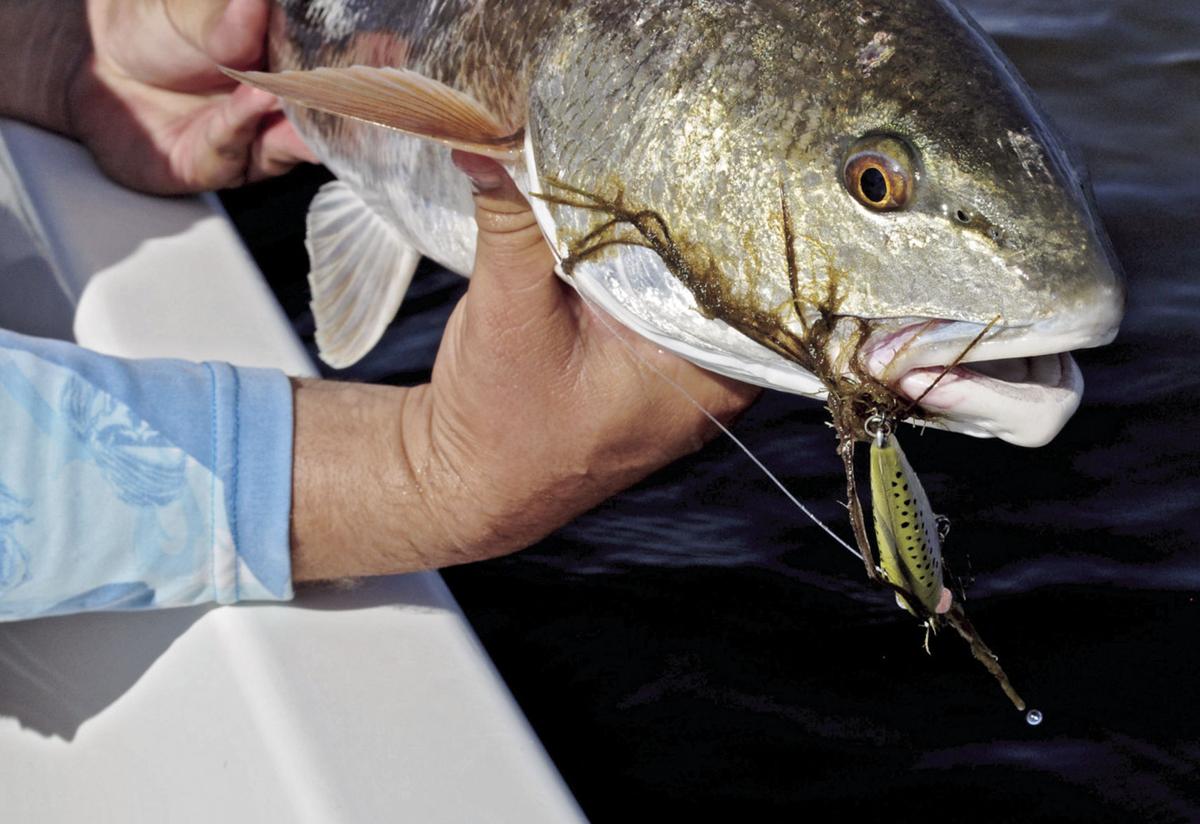In this realistic, close-up outdoor photograph, a person in a long-sleeved blue shirt is holding up a large, freshly caught fish. The fish, which is silvery-gray with a white belly and a black eye, has its mouth open, revealing a hook lodged at the corner with a green, black-spotted bait in its mouth. The person's hands are coming from both sides of the image, resting on the edge of what appears to be a white boat, contrasting against the dark blue or black rippling water in the background. Only the person's arms are visible, emphasizing the impressive size of the fish.